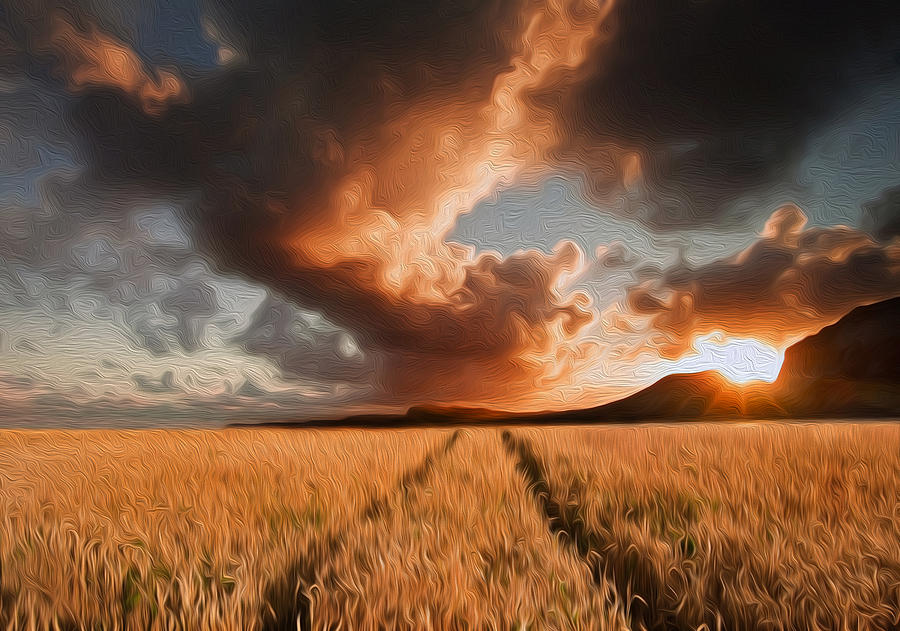This image, reminiscent of Van Gogh's "Starry Night," vividly depicts a lush wheat field extending into the horizon beneath a dramatic, swirled sky. Dominated by large, uneven brushstrokes and circular patterns, the artwork conveys a sense of motion and texture throughout. The golden wheat, waving like strands of blonde hair, is divided by two tire tracks that stretch endlessly towards a distant mountain range. Above the mountains, which stand silhouetted against the horizon, the vibrant sun prepares to set, casting beams of light from a jagged shape partially obscured by thick, dark clouds with gradients of blue to gray. These clouds, interspersed with white streaks, add to the complexity and depth of the sky, swirling and blending with the overall color scheme of brown and gold fields. The captivating sunset amplifies the painting’s ethereal quality, embodying the artist’s intricate manipulation to highlight the dynamic interplay between the earth and the heavens.